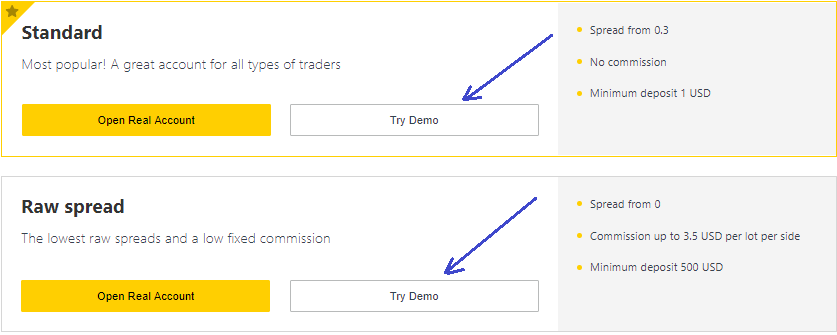In this image, there are two distinct rectangular sections, each containing specific information. 

At the top, the rectangle features a yellow corner with a star icon and the label "Standard," accompanied by the text "Most Popular - A great account for all types of traders." Below this, there is a prominent yellow rectangle with black text reading "Open Real Account." Next to it, a white box offers an option to "Try Demo." A digitally drawn blue arrow directs attention towards the "Try Demo" option.

Adjacent to this, and framed with a gray background, three bullet points highlighted in yellow list key features: "Spread from 0.3," "No Commission," and "Minimum Deposit 1 USD."

The bottom rectangle is labeled "Raw Spread," detailing it as offering the "Lowest raw spread and a low fixed commission." Similar to the top section, this area also includes buttons for "Open Real Account" and "Try Demo," with a digitally produced navy arrow emphasizing the "Try Demo" option.